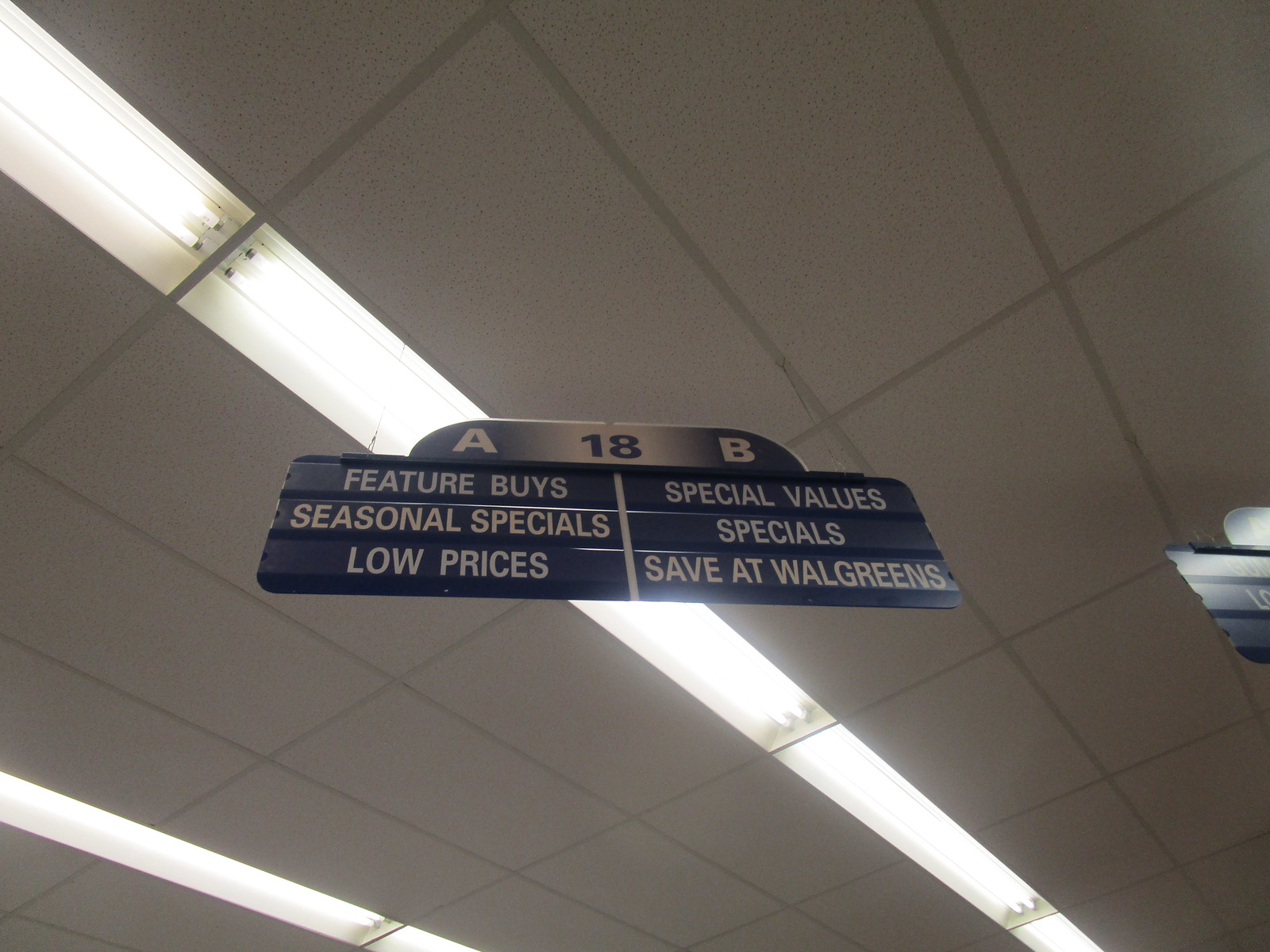This photograph, taken inside a store, captures one of the aisle signs. The camera angles upward towards the ceiling, centering the sign prominently. The sign's header features the letter "A" at the top left with "18" in the center, and "B" on the top right. Beneath the "A" section, the text reads "Feature Buys, Seasonal Specials, and Low Prices," while the "B" section states "Special Values, Specials, Save at Walgreens." The sign itself is blue with white lettering. Above, the ceiling is visible with rectangular ceiling tiles and a couple of strips of lighting.